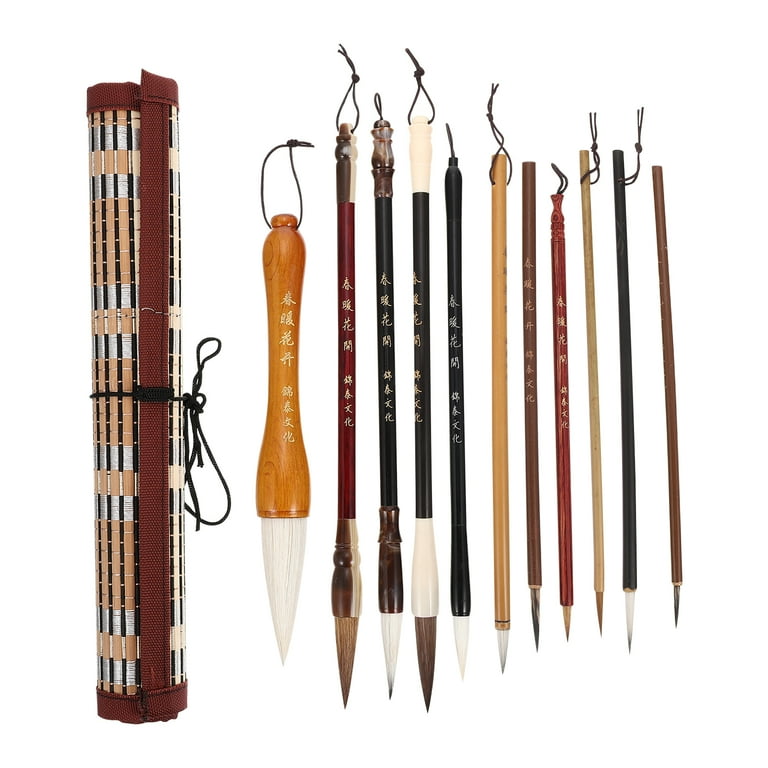This image showcases a detailed calligraphy brush set consisting of 11 brushes, each with a distinctive wooden handle adorned with Japanese writing. The brushes range in size from large, thick-bristled brushes to very thin ones, similar to pencils. The largest brush features a natural wood handle and a densely packed white triangular head. Following this, there’s a smaller red brush, succeeded by several thin brushes in various shades like light brown, dark brown, and black. All brushes carry intricate Japanese characters, enhancing their traditional aesthetic.

To the left of these brushes is a rolled-up bamboo case, resembling a small tatami mat. The bamboo slats are held together by silver threading and bordered by maroon piping, giving it a refined finish. This case is tied securely with a black string, allowing it to roll up neatly into a compact tube. This elegant storage solution provides both protection and portability for the calligraphy set. The harmonious combination of natural materials and traditional craftsmanship makes this calligraphy brush set both functional and beautiful.